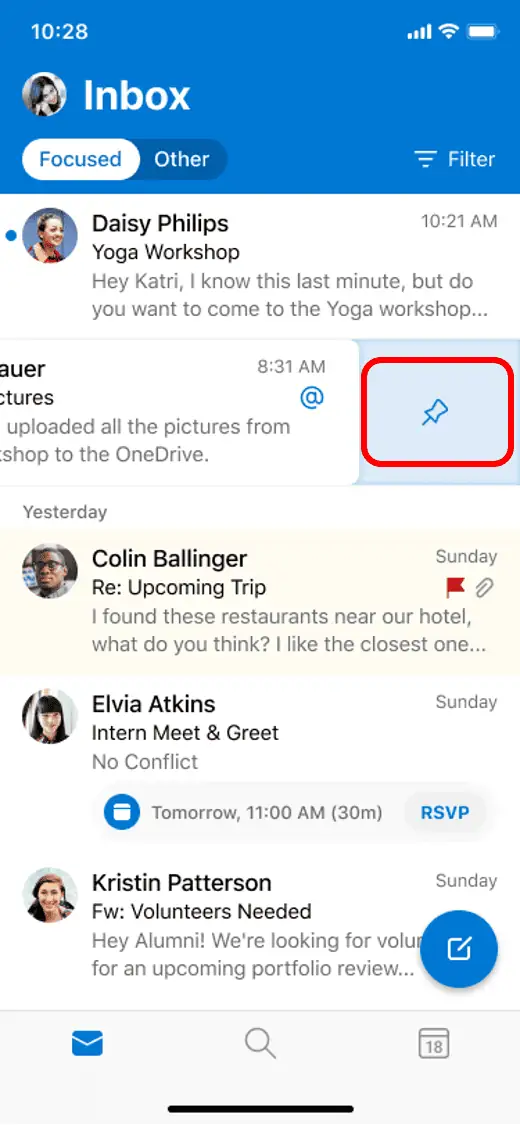**Detailed Caption for the Image:**

The image is a portrait-mode screenshot of an email inbox, with a specific section highlighted in a red border for emphasis. The topmost part of the screenshot displays a light blue band stretching from the upper left to the upper right corner. Within this band, the time "10:28" is visible, along with a full battery icon, indicating a well-charged device.

Just below this, a navigation bar displays the label "Inbox" and features a circular avatar of a person with black hair, seemingly a female. Beneath this bar, there are two distinct tabs labeled "Focused" and "Other." The "Focused" tab appears as a white button, while the "Other" tab is a darker blue button, indicative of its active status. Additionally, there is a filter option for email categorization on the right side.

The first email listed is from Daisy Phillips regarding a "Yoga Workshop." The subject line reads, "Hey Katri, I know this is last minute, but do you want to come to the yoga workshop?" This email is timestamped at "10:21 AM."

Scrolling down, another email is partially visible, especially due to the presence of a large red circle drawn around a pushpin icon on the right side, signaling its importance. The subject of this email reads, "Uploaded all the pictures from shop to the OneDrive," and is timestamped at "8:31 AM."

Further emails listed include:
- An email from Colin Ballinger about an "Upcoming Trip," discussing restaurant options near a hotel, marked with a red flag.
- An email from Elvia Atkins regarding an intern meet-and-greet scheduled for "Tomorrow at 11 a.m." with an indication of "No conflict" and a highlighted note that it's a "Sunday."
- An email from Kristen Patterson Peterson titled "Forward: Volunteers needed," calling for alumni volunteers for an upcoming portfolio review, and featuring a blue edit button on the right of the message.

These highlighted and circled elements within the red-bordered section suggest key information and activities planned, aimed to draw specific attention to these details.